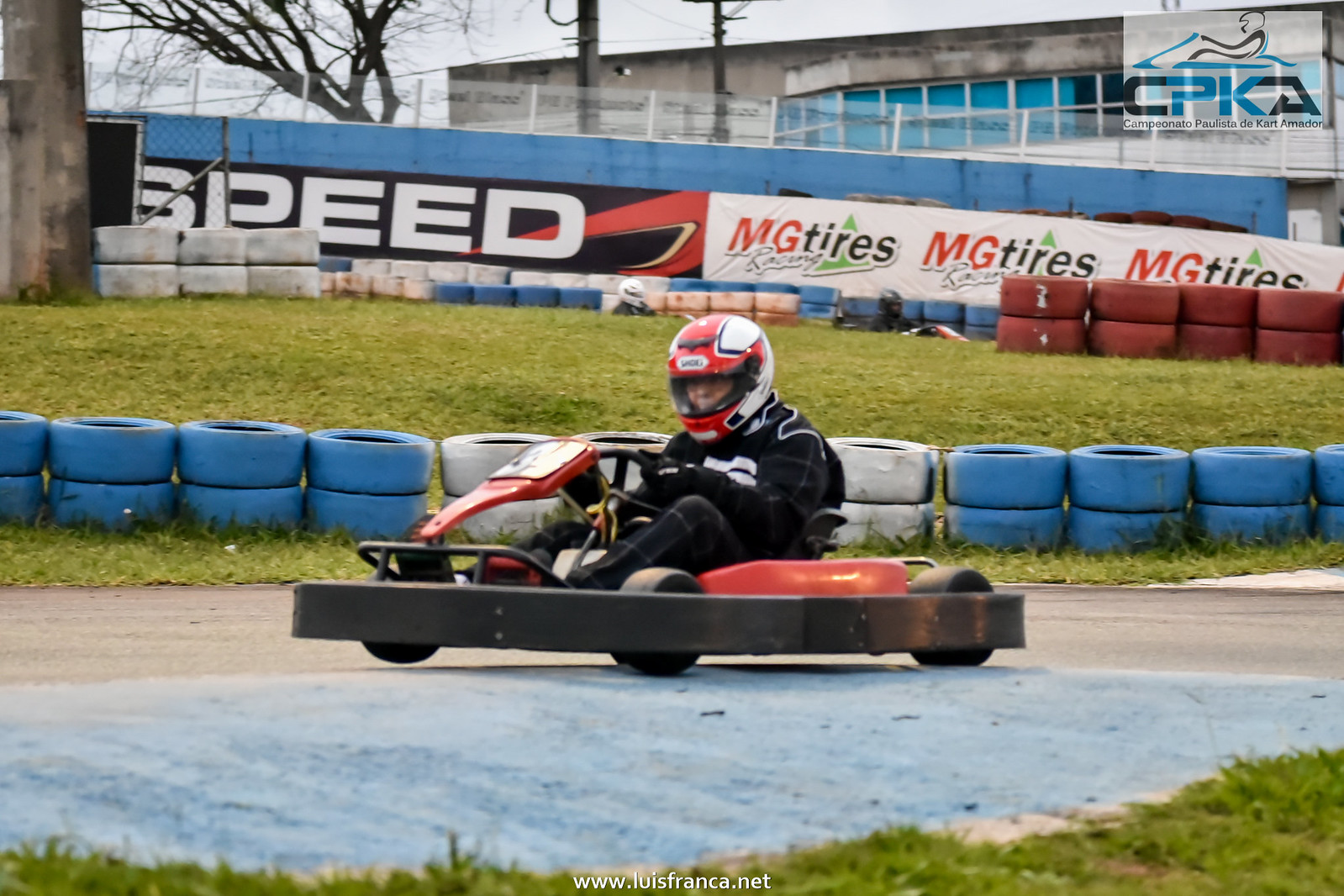The image captures a dynamic outdoor scene featuring a go-kart racing on a concrete track. At the center, a driver wearing a red and white full-face helmet with a visor, and a black and gray racing suit with white trim, maneuvers a low-to-the-ground red and black go-kart. The front and sides of the go-kart are predominantly red, with a black steering wheel and a protective black bar encircling the vehicle. The driver’s legs and knees straddle the go-kart, emphasizing its compact design. 

The setting is a mix of natural and artificial elements, starting with a grassy field at the bottom of the image that transitions into a concrete track marked with blue lines. Surrounding the track are green grassy hills adorned with blue, white, and red tires that serve as barriers. Several buildings with concrete facades and blue-framed windows populate the background, along with wooden poles and a leafless tree, suggesting a structured but open outdoor environment.

Multiple advertisements and banners are visible along the top of the image and on a blue wall to the right. Notable among them are “MG Tyres” with red and black text, and “Speed” in white on a black and red background. The top right corner features a logo with "CPQA" and an outline of a go-kart, representing the "Campeonato Polista de Dakar Amador." Additionally, white text at the bottom of the image spells out “www.luisfranco.net,” providing information about the event or the photographer. The overall palette includes red, black, white, blue, green, gray, brown, yellow, and tan, enhancing the vividness and energy of the racing scene.